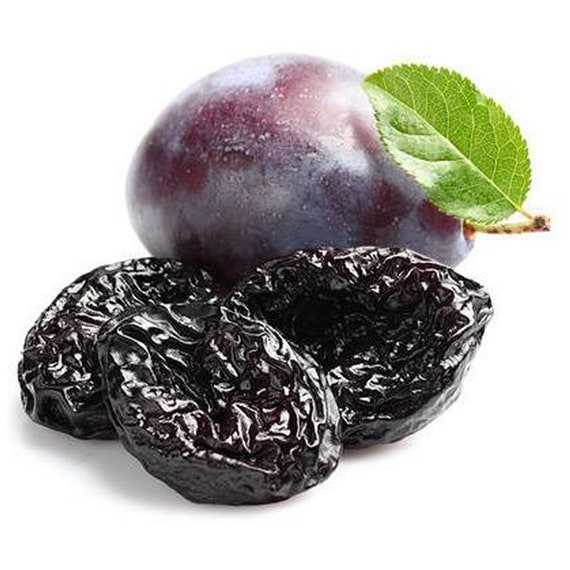The image is a professional photograph featuring a purple plum and three prunes on a white background. The plum, positioned at the back, is a rich purple color with a brown stem oriented to the right. Attached to the stem is a small, bright green leaf with finely serrated edges and a prominent central vein, pointed towards the middle of the plum. The plum exhibits a glossy surface with light reflections, giving it a slightly frosted appearance with hints of white and silver, suggesting a dewy freshness. In front of the plum, three prunes, dark and nearly black in color, are artfully arranged in a slightly overlapping triangular pattern. The prunes display intricate wrinkled ridges and are softly shadowed underneath, enhancing their textured appearance against the pristine white background, which appears meticulously clean and unaltered.